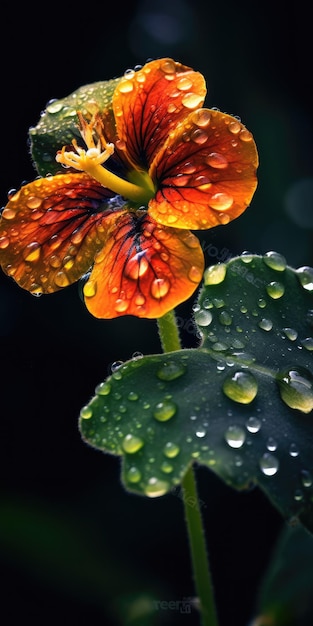This close-up photograph captures a striking orange flower with five slightly rounded petals, four of which boast subtle hints of green along the edges and dark blue veins. The flower features a yellow cylindrical stamen at its center, sprouting into multiple filamentous ends reminiscent of a sea anemone. The bloom, adorned with numerous droplets of dew or rain, sits on a thick, light green stem. Surrounding it are green leaves, also dotted with water droplets, with some in front of the flower appearing slick and dark green, almost butterfly-shaped. The flower appears to face towards the camera and slightly angled to the left. The entire scene is set against a solid, black backdrop that dramatically enhances the focus on the glistening, moist plant in the foreground.